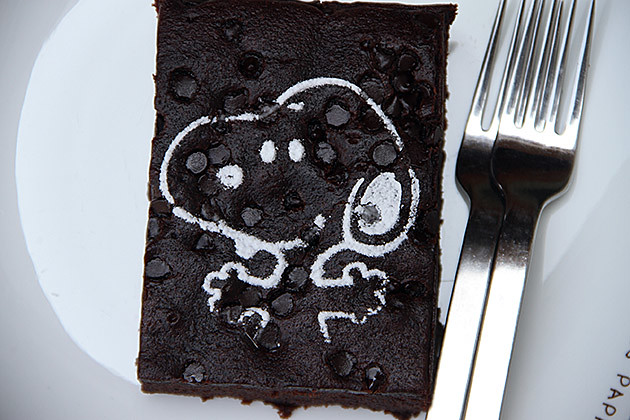In this wide rectangular photograph, we are looking down onto a white plate that is approximately five inches wide and three inches tall. The plate features a slightly off-white background with a grayer border on the left side and the bottom right corners, creating a subdued framing effect. At the center of the plate sits a tall rectangular piece of dessert, which appears to be a rich chocolate brownie, distinguished by its dark, almost black top surface studded with mini chocolate chips. Adorning the top of the brownie is an intricately stenciled white outline of Snoopy, the beloved cartoon dog. Snoopy’s head faces left, with his signature large oval eyes close together, and his arms extended outwards. The image of Snoopy is likely made using powdered sugar. To the right of the brownie, two silver forks are positioned, with one fork neatly overlapping the other. In the bottom right-hand corner of the plate, partial handwriting can be seen, displaying the letters "PAP." The plate also exhibits a subtle glare on the left, forming a circular light effect that slightly darkens the upper and lower left and right corners of the plate.